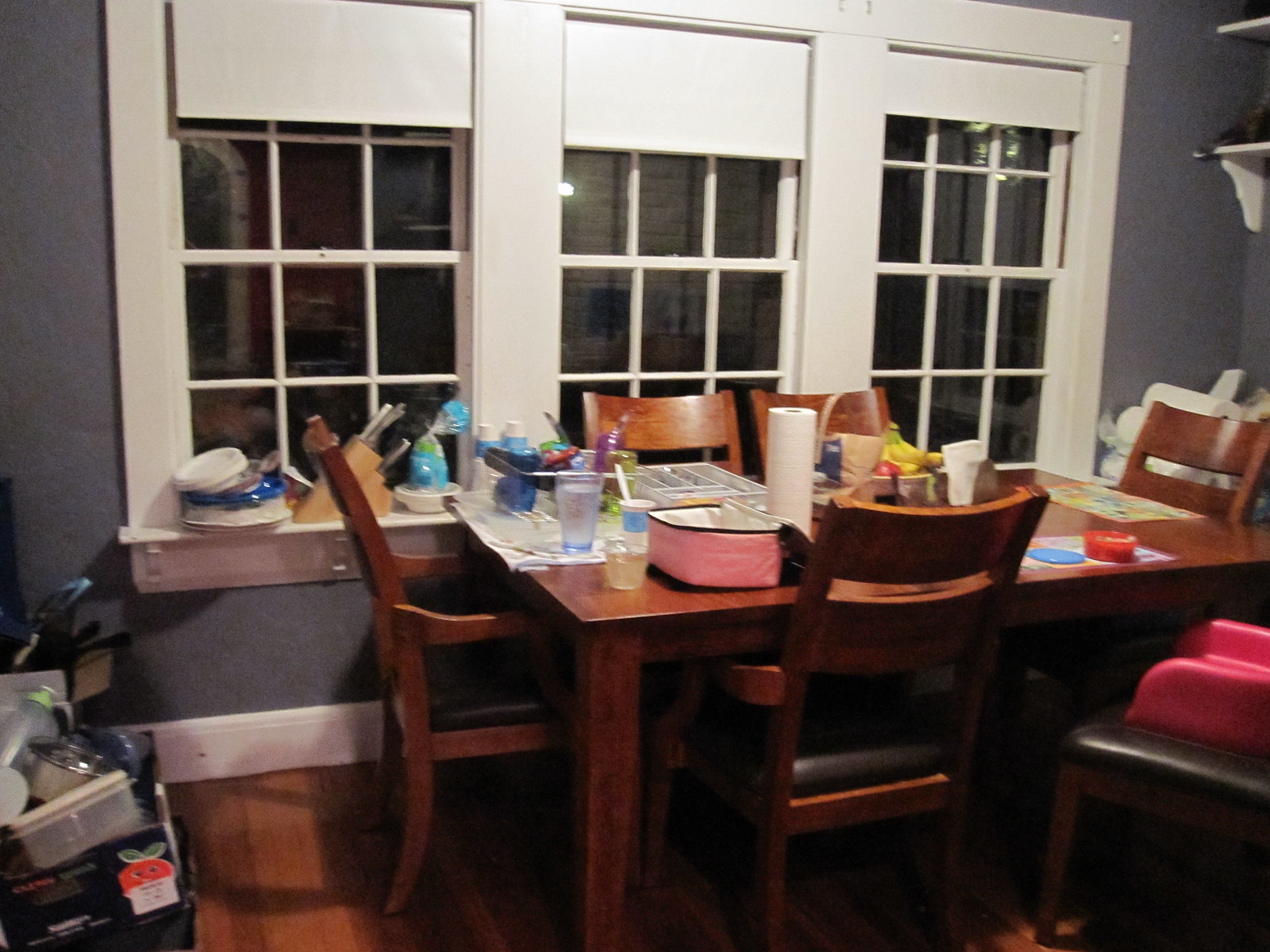In this photograph of a cozy living room, the back wall is painted a dark gray, providing a dramatic backdrop. Centrally positioned on the wall are three windows, each framed with a crisp white border and capped with small, nearly closed white blinds. The first window on the left has its sill adorned with a few dishes and a wooden block containing knives. In front of the remaining two windows stands a sturdy rectangular wooden table, surrounded by six chairs—one at the head, one at each end, and two along each side, each equipped with a placemat.

Notably, the chair in the bottom right-hand corner is pulled out, revealing a black cushion topped with a red booster seat for a child. Scattered across the table, a roll of paper towels sits at its center, suggesting ongoing activity or a recent meal. On the left side of the table, two glasses can be seen—one blue and one clear—accompanied by a cup of yogurt with a plastic spoon, indicating a casual, lived-in warmth.